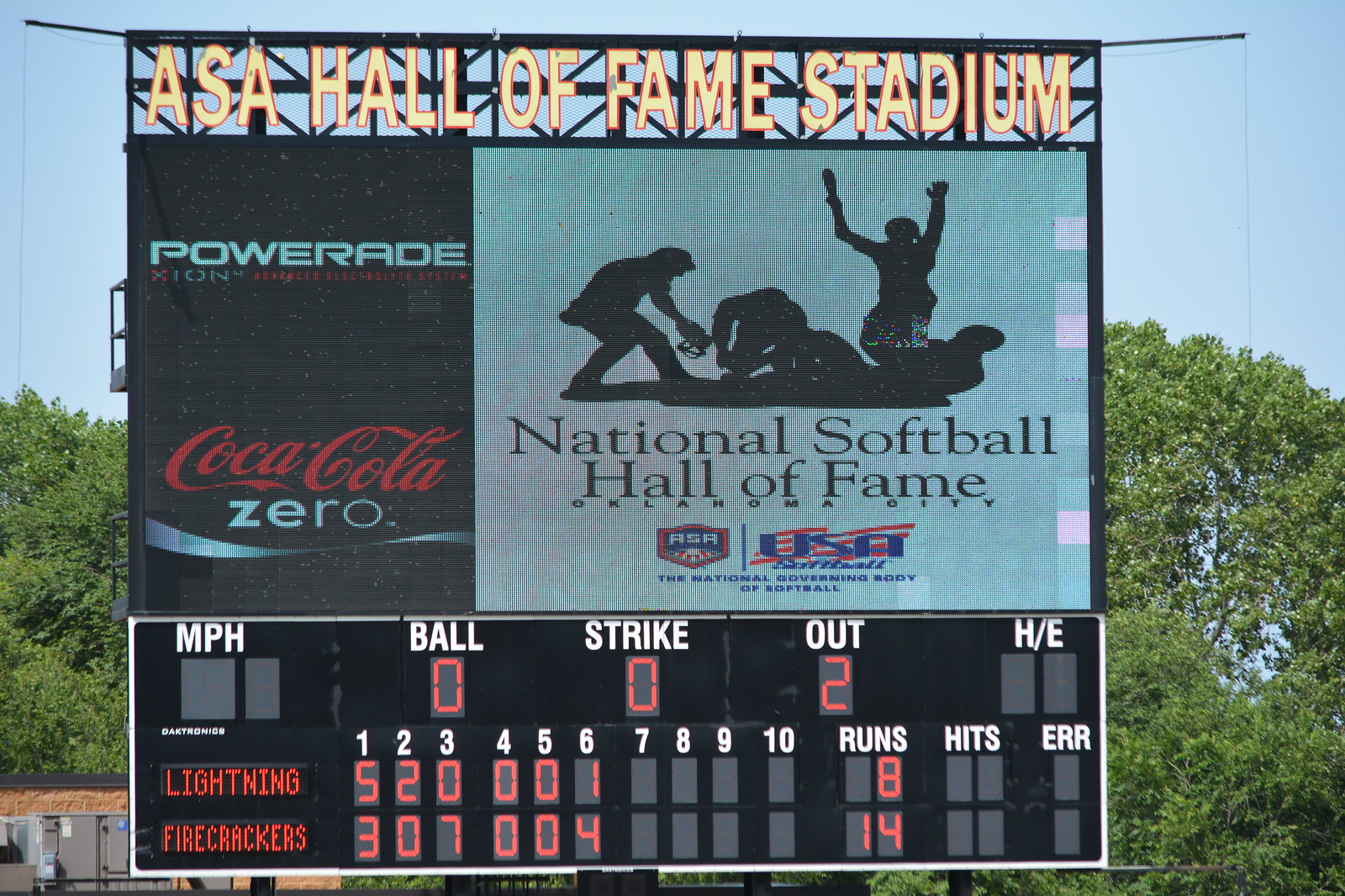This is a detailed image of the ASA Hall of Fame Stadium scoreboard, set against a backdrop of lush trees and some visible power equipment. At the top of the scoreboard, the gold-lit letters spell out "ASA Hall of Fame Stadium." Below, on the left-hand side, are advertisements for Powerade and Coca-Cola Zero. Adjacent to these ads is a large light blue square featuring black silhouettes of softball players and the words "National Softball Hall of Fame Oklahoma City."

The main section of the scoreboard displays the game's status. Across the top, white letters indicate various game metrics: "Miles per Hour," "Ball," "Strike," "Out," and "H/E." The scoreboard shows that the Lightning are playing against the Firecrackers, with the Lightning currently trailing. The Lightning have scored 8 runs while the Firecrackers lead with 14 runs. The scoreboard also shows that the count is zero balls, zero strikes, and there are two outs. The numbers one through ten across the top track inning-by-inning scores, and the columns for "Runs," "Hits," and "Errors" provide additional game statistics. The scene is illuminated by natural light, suggesting it's daytime or early evening.